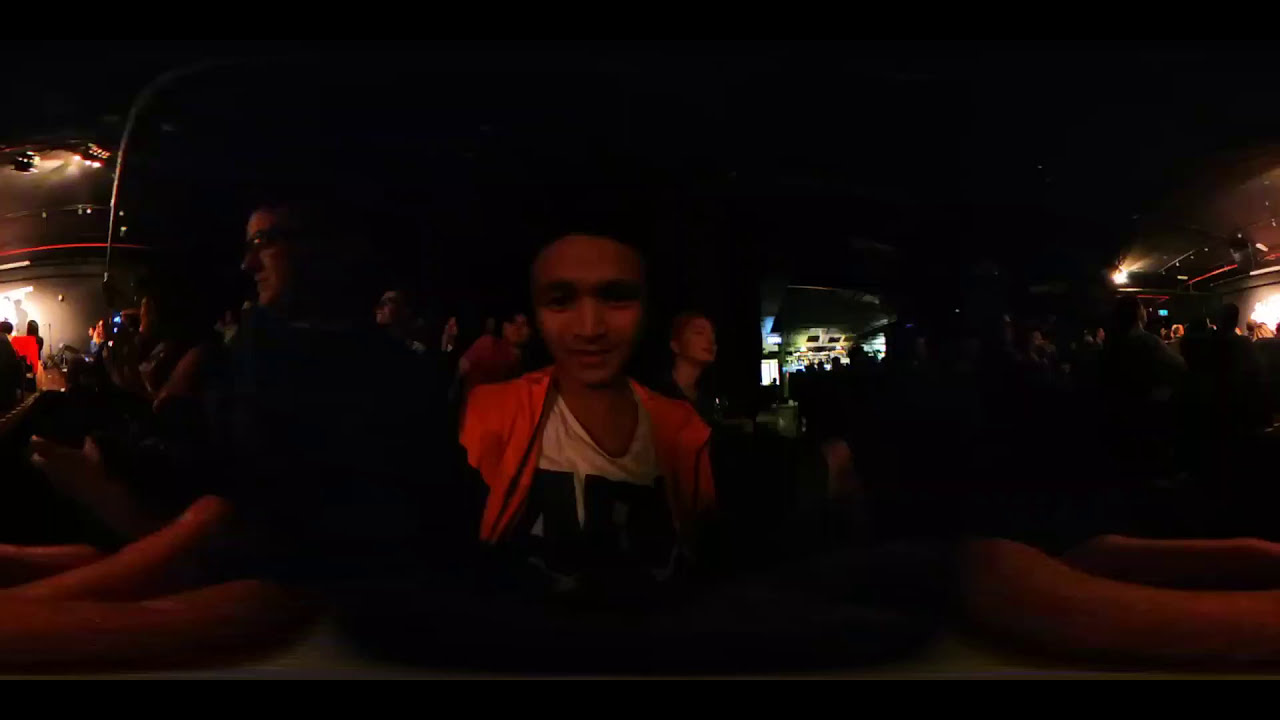In this indoor photograph taken in a very dark room, the center of the image prominently features the upper torso and head of a young man with darker brown skin, possibly of Asian descent. His face is illuminated by a reddish glow that graduates from a pale forehead down to a darker chin. He is dressed in a white t-shirt with black print, over which he wears a reddish-orange jacket. 

Flanking him are two individuals with fair skin also cast in the same reddish light, one of whom is a tall man with glasses standing to his right and slightly behind. The left and right edges of the photograph are primarily shrouded in darkness, save for bright spots where lights reveal a large, crowded room, possibly a bar, filled with people who appear to be looking up towards a stage. The image effect gives a surreal impression, as if parts of the scene, particularly what may be the man's outstretched arms, morph into octopus-like limbs disappearing into the dark. A long table obscured by shadows is discernible in the foreground. A sense of a crowded, almost chaotic atmosphere pervades the image, underlined by the juxtaposition of silhouettes bathed in intermittent red light.